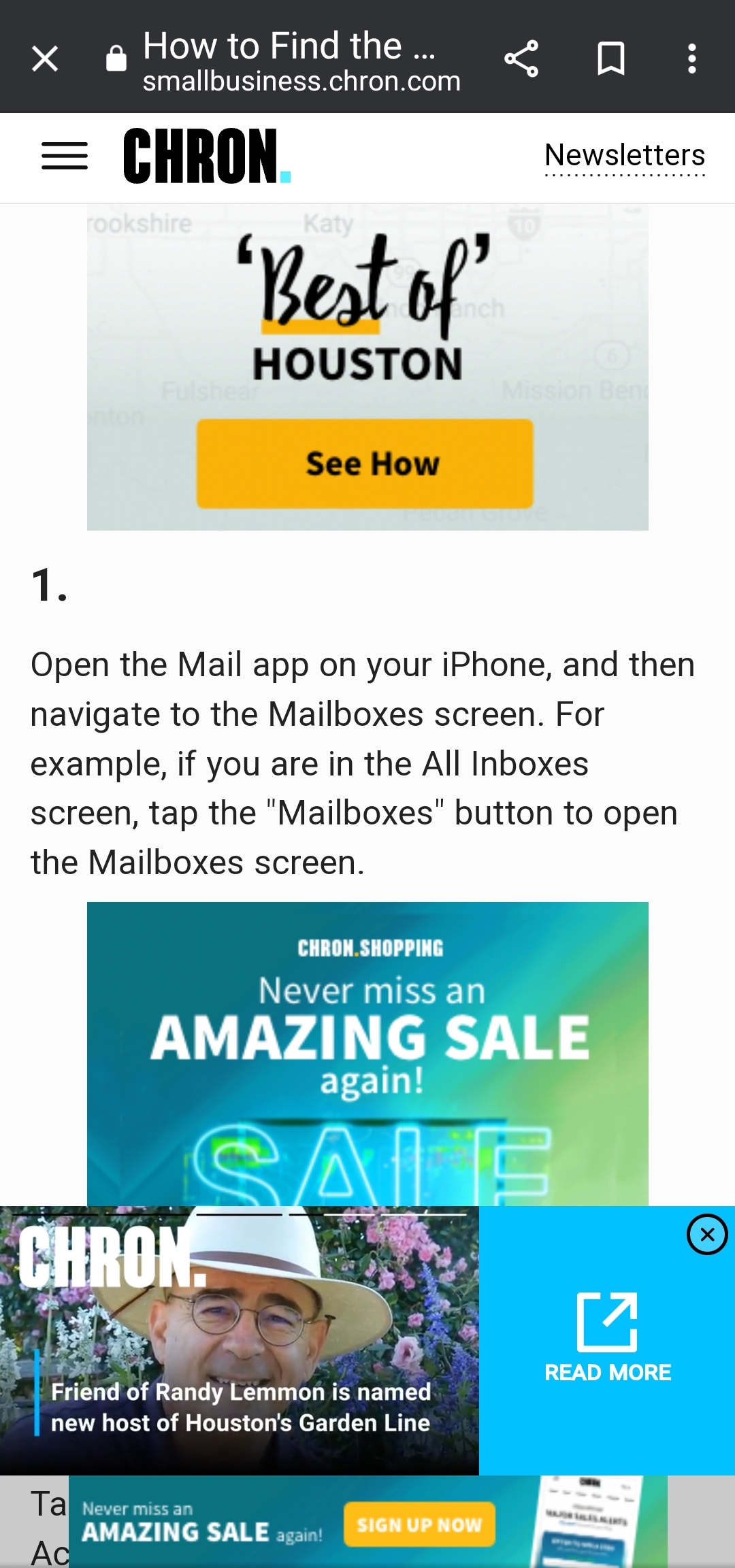This image features a webpage from smallbusiness.cron.com, as evident from the URL displayed at the top center of the screenshot. The webpage header includes a black box on the left with an "X" button and the text "How to find..." in the middle. Below the URL, "C-H-R-O-N" is prominently displayed in bold, black capital letters. Adjacent to this, there is a "Newsletters" link.

Next, the main content area starts with a gray box titled "Best of Houston," with the word "Best" underlined in yellow. Beneath this box, there is a yellow button labeled "See How" in black letters.

The instructional content follows with the text: "1. Open the Mail app on your iPhone and navigate to the Mailboxes screen. For example, if you're in the All Inboxes screen, tap the Mailboxes button to open the Mailboxes screen."

At the bottom of the screenshot, there's an advertisement with a turquoise-greenish background that reads: "Cron Shopping - Never miss an amazing sale again."

This webpage provides detailed instructions on navigating the Mail app on an iPhone, with a clear layout and supplementary advertisements.